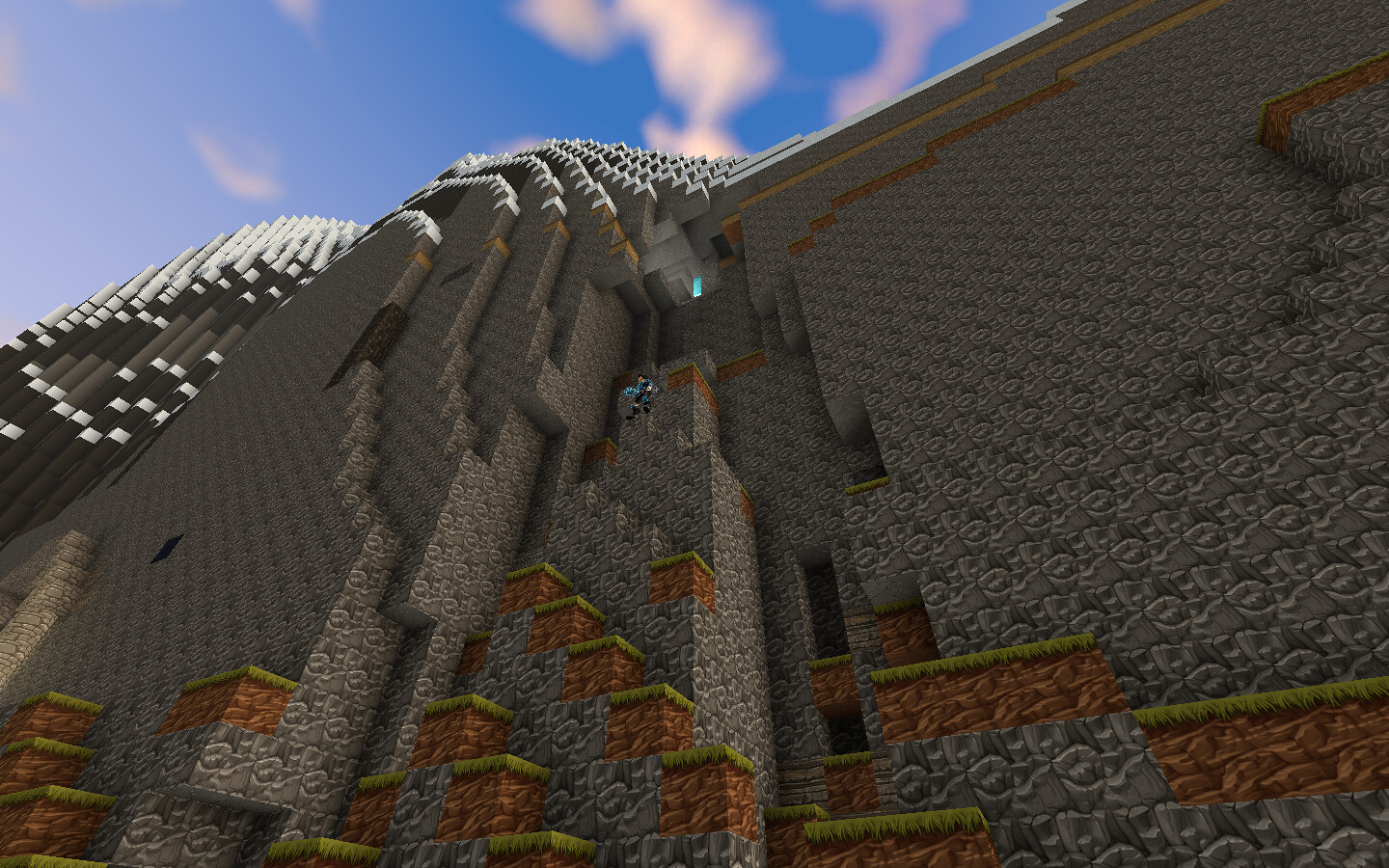This vibrant color photograph appears to capture a scene from a video game with a predominant dark taupe color palette accented by vivid orange and yellow hues. A human figure stands out in the foreground, dressed in a blend of turquoise, black, and gray, with white skin and jet-black hair adding contrast. The figure seems to be part of a larger structure resembling a building or possibly a mountainside constructed with elements that evoke Lego-like bricks. The steps of this structure are painted orange with yellow edges, while the main body is rendered in dark taupe, capped by a lighter white section at the top. The scene is set against a backdrop of a partially cloudy sky, with puffy white clouds congregating towards the center where the sky is a deeper blue. The left side of the sky is lighter, almost cloudless, creating a dynamic contrast. The overall impression is one of a whimsical, blocky environment suggestive of a video game, though the exact nature of the game remains unclear.